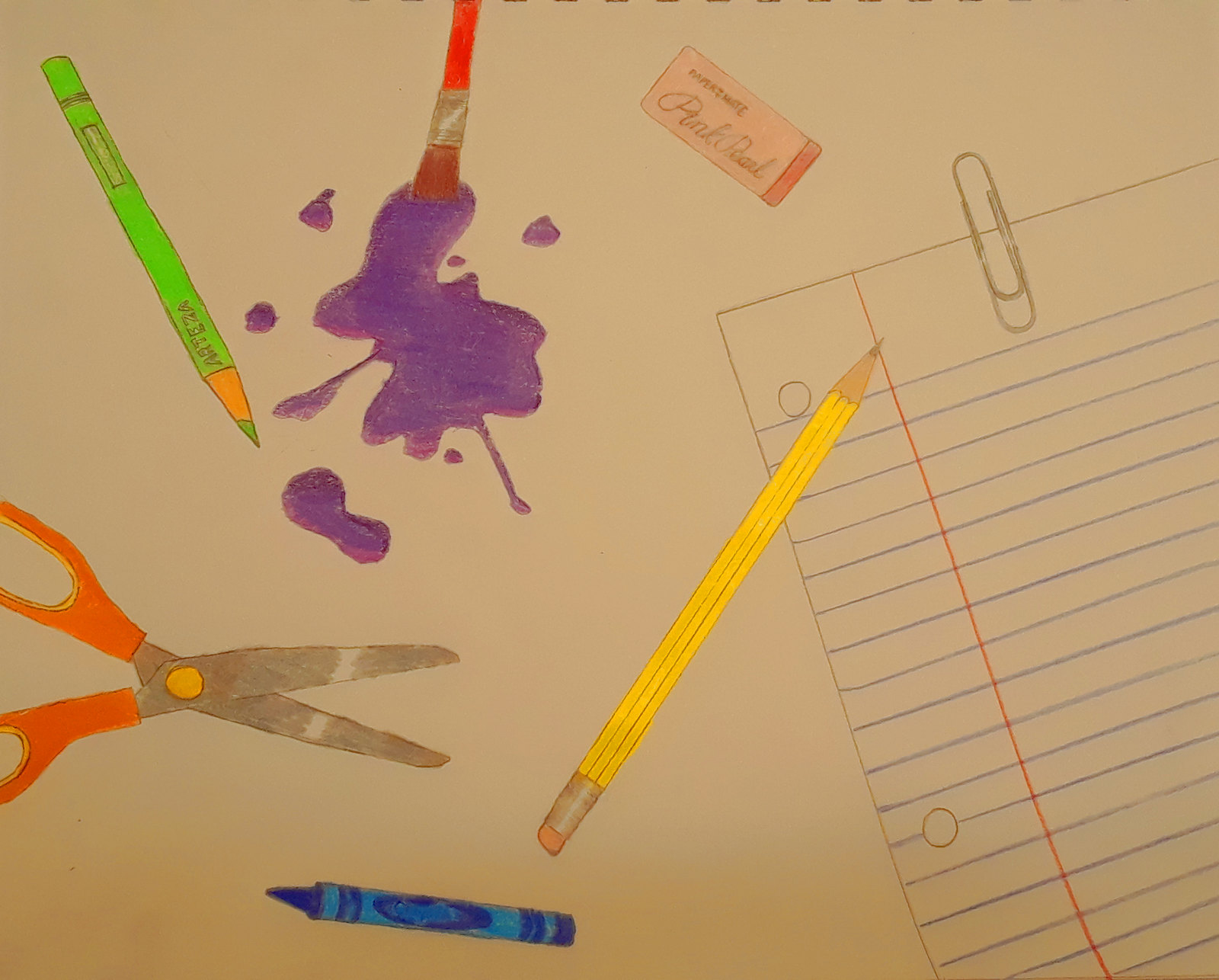This drawing depicts a cluttered yet creative young person's workstation. On the right side of the picture, you see wide-ruled notebook paper angled slightly to the left, secured with a paperclip. Resting on top of the paper is a yellow pencil with a pink eraser at its end. Scattered across the workspace are various art supplies: a green colored pencil, a blue crayon, and a pair of scissors with orange handles. Towards the center of the image, blotches of purple paint are evident, suggesting a spill, with a small paintbrush with an orange handle left amidst the mess. Additionally, a classic rectangular pink eraser, reminiscent of school days, sits near the top of the image. These elements collectively illustrate the tools and potential chaos of a budding artist’s creative process.